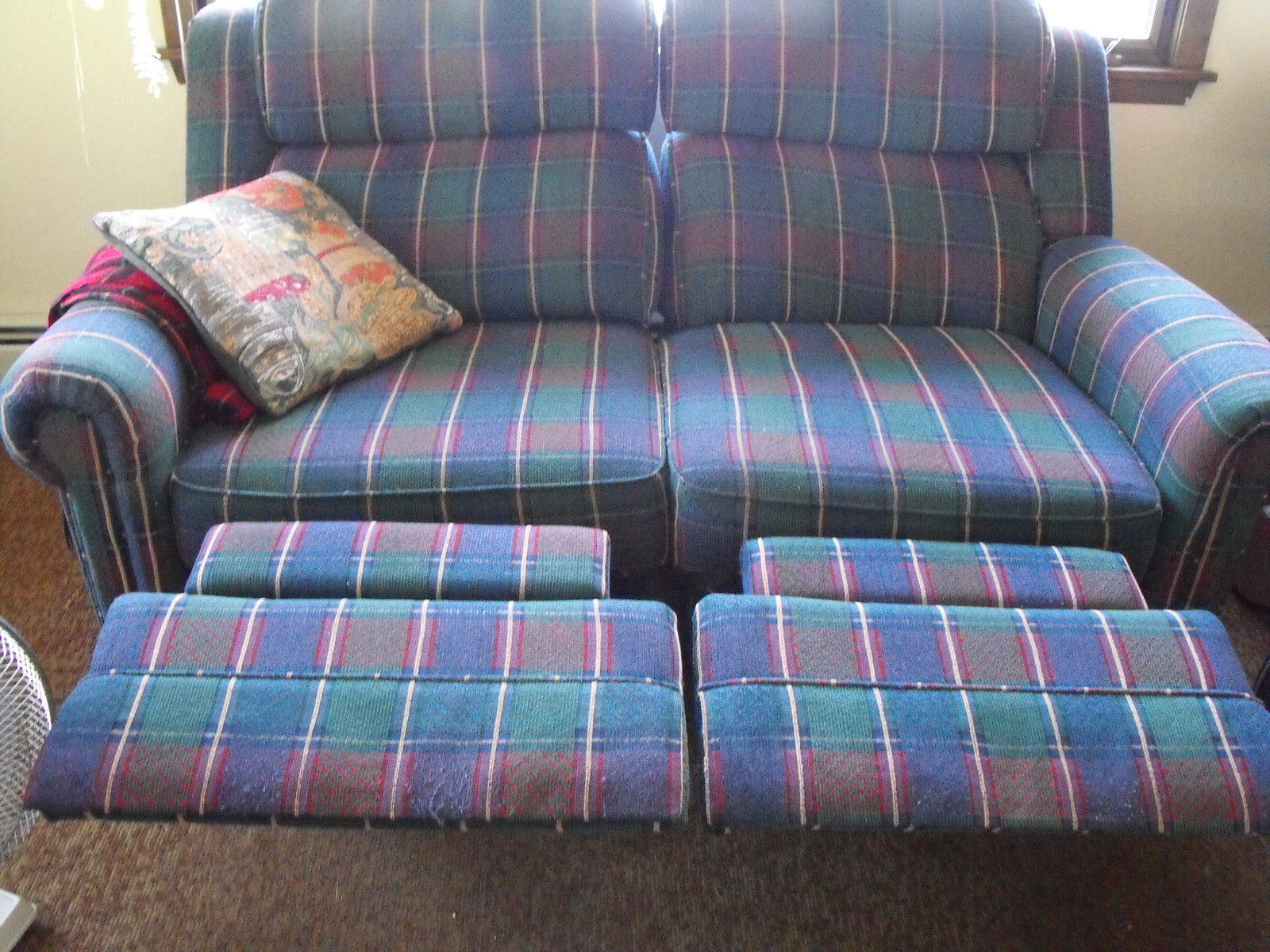The image depicts a well-worn plaid reclining loveseat with prominent blue, green, and red stripes separated by white lines, creating a vivid yet coherent pattern. Both seats are in a reclined position, displaying raised footrests. Draped over the left armrest is a red and black plaid blanket, adding a touch of warmth and homeliness to the setting. The loveseat features an embroidered pillow with a fruit motif, including images of corn, oranges, and tomatoes, placed near the armrest, and a hint of a pink blanket or coat beneath it. Positioned on brown carpet, the loveseat sits in front of a sunlit window framed in either black or wood, partially obscured by the angle of the photo. In front of the loveseat, to the left, there is an oscillating fan visible, suggesting a cozy and lived-in environment ready for sale.